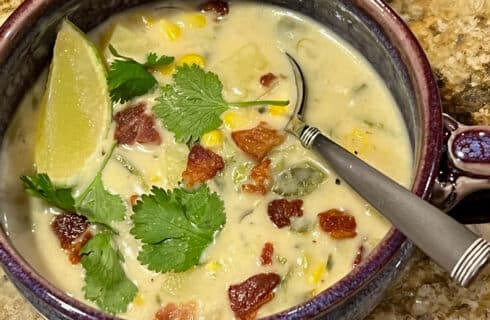This image features a bowl of creamy potato corn chowder, prominently placed on a brownish-yellow and cream granite countertop. The brown bowl, equipped with a handle, contains chunks of potato and vibrant yellow corn kernels, interspersed with visible hints of green chilies. A crispy layer of bacon and a sprinkle of fresh green cilantro adorn the top of the chowder, adding both texture and color. A decorative silver spoon rests inside the bowl, while a fresh lime wedge lies to the left, completing the presentation.